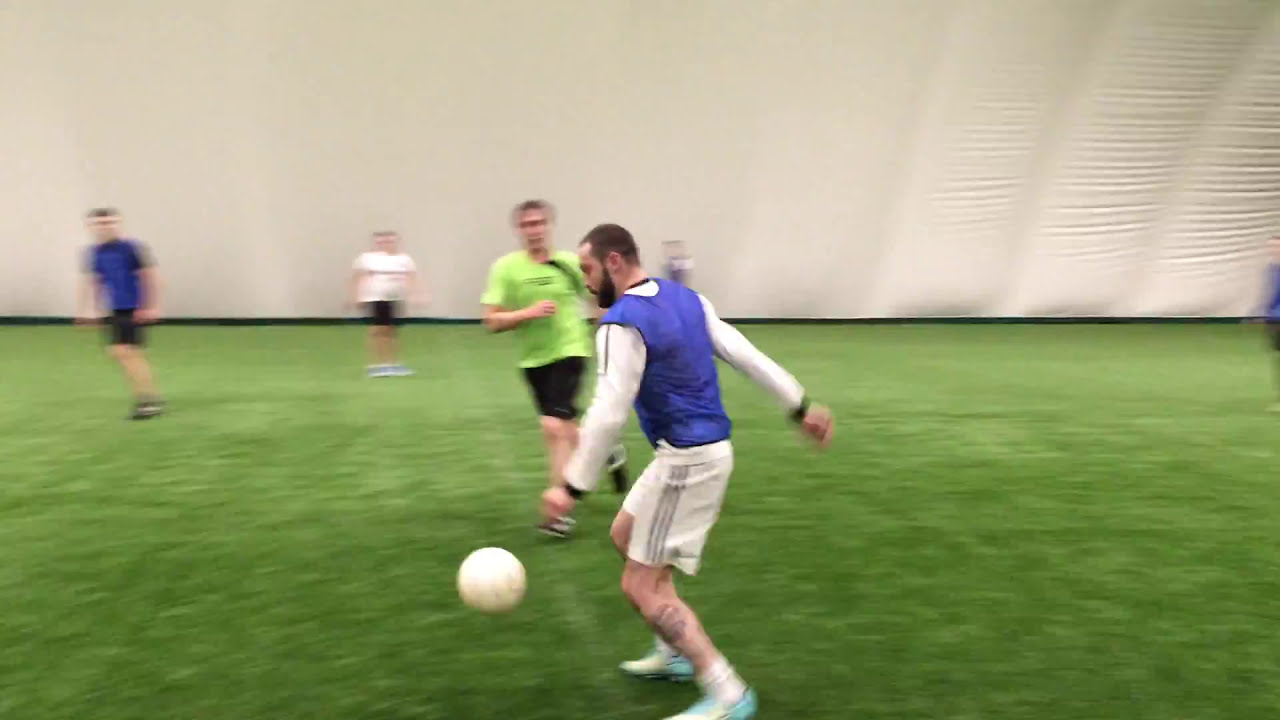In this detailed action photograph, there are several men playing soccer on a bright, lush green grass field, which is situated indoors under a large white-walled or tarp-covered structure. The central focus is a man in the foreground wearing a distinct uniform: white shorts with three black stripes on the side, a white long-sleeve shirt beneath a blue sleeveless vest, white socks, and light-colored athletic shoes. He has tattoos on his legs and sports dark brown hair and a full beard. His stance and the position of his extended arms suggest he is about to kick the white soccer ball near his legs.

To his right, a man in black shorts and a neon green t-shirt is running towards the ball. This man has lighter brown hair and no beard. In the background, the images of several other players are blurrier due to motion. One of these players wears black shorts and a white t-shirt, while another is clad in black shorts and a dark blue t-shirt, both of whom are at a greater distance. All the players appear to be Caucasian. The right side of the image reveals more of the flat green field along with the white background, highlighting the indoor setting of this vibrant, dynamic scene.